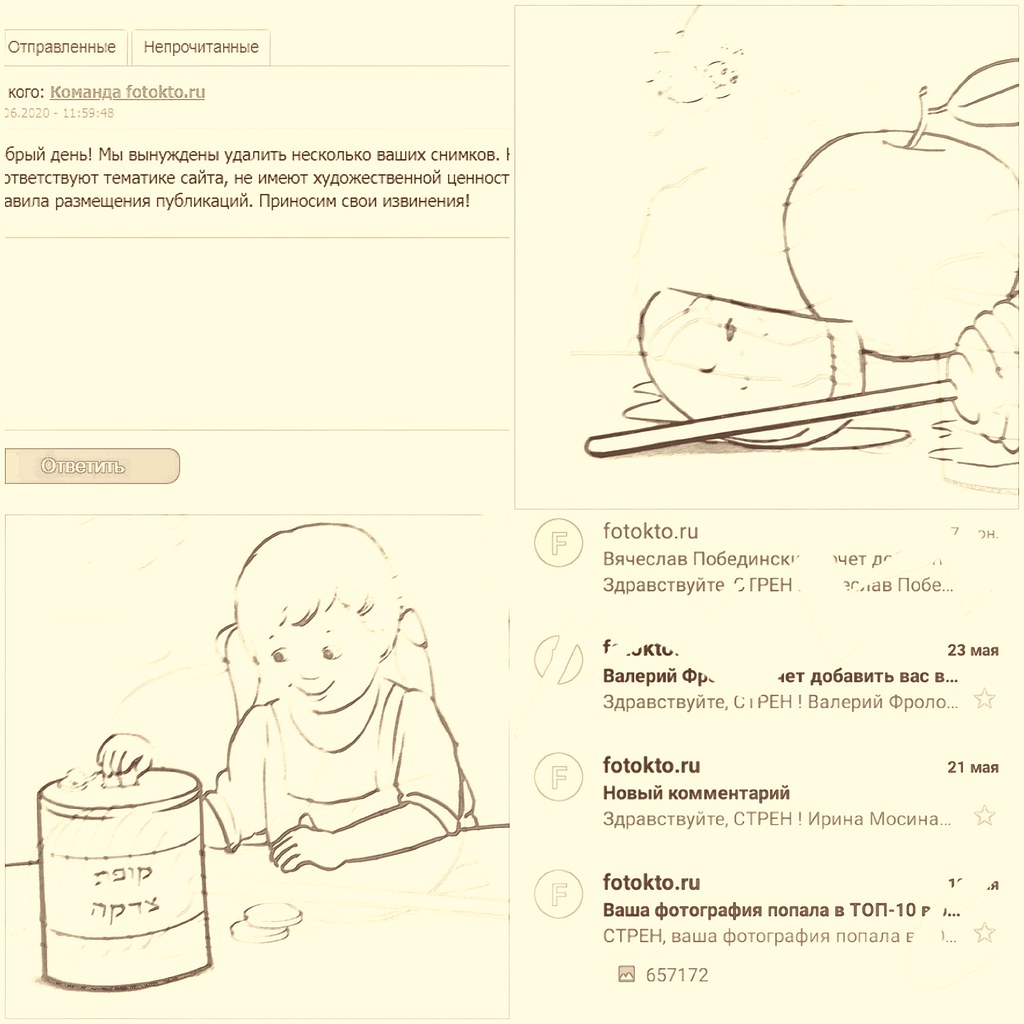In this illustrated image with a pale yellow background, the content is divided into two columns. The text appears to be in a language that could be Russian, Japanese, or Ukrainian, with a consensus leaning towards Russian. On the left-hand column, there are two tabs at the top labeled in this language, with some information provided under these tabs. Below this information, there's a white space followed by a clickable button, and further down, a lightly sketched drawing of a young girl in black ink. The girl is reaching into a cylindrical object, possibly a cookie jar or perhaps a piggy bank, with a smile on her face, wearing pigtails and a t-shirt.

In the right-hand column, the top features a sketched image of various fruits, including an apple, a slice of another fruit, and a honey stick. The details of these sketched illustrations are minimal, emphasizing just the outlines. Beneath this fruit illustration, there appears to be a list of menu items accompanied by their prices, all written in the same foreign language, suggesting that the image may depict a page from a menu or a website with a social media-like interface. Additionally, there are words “photocto.ru” and a date "2020 11 59 48" suggesting some sort of timestamp or watermark typically found in digital content.